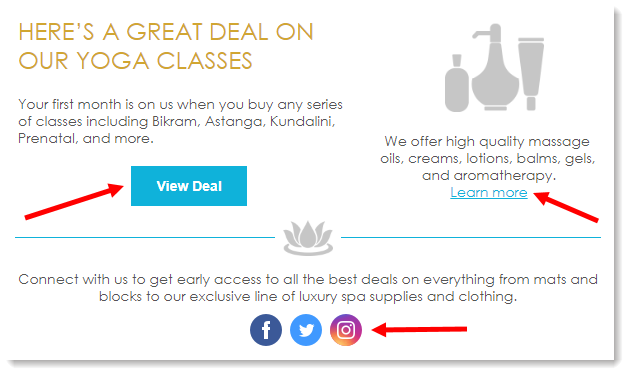**Caption:**

In this vibrant, yellow-toned promotional image, we invite you to take advantage of an amazing offer on our yoga classes. Prominently displayed on the right is a sleek graphic design featuring a collection of wellness products, including a large oil decanter with a pump, a bottle, and a lotion container.

The text announces: "Here's a great deal on our yoga classes. Your first month is on us when you purchase any series of classes, including Bikram, Ashtanga, Kundalini, Prenatal, and more." 

Below this enticing offer, there is a distinct blue rectangular button labeled "View Deal," highlighted by a red arrow pointing towards it.

In addition, the image promotes our high-quality range of wellness products: massage oils, creams, lotions, balms, gels, and aromatherapy items. A "Learn More" link, also blue and underlined, comes with a red arrow pointing to it.

Central to the design is a delicate lotus flower graphic flanked by blue lines, emphasizing the holistic nature of our offerings. Accompanying text reads, "Connect with us to get early access to all the best deals, including everything from mats and blocks to our exclusive line of luxury spa supplies and clothing."

Finally, social media icons for Facebook (blue), Twitter (light blue), and Instagram (a gradient of yellow, red, and purple) are placed at the bottom right. Each is highlighted by red arrows, encouraging you to stay connected with us online.